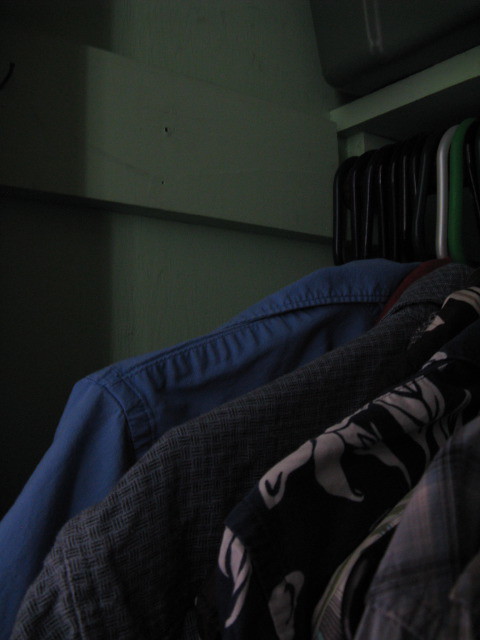The image depicts an indoor setting, likely a closet, featuring a collection of collared button-down shirts hanging on black hangers. The backdrop consists of a plain white wall to the left and a green-painted wooden closet with a shelf extending from the center to the upper right corner. The shirts are the primary focus and are centrally positioned in the image. Starting from the left, there is a royal blue collared shirt, followed by a dark gray, almost purple checkered shirt. Next, there is an Aloha style shirt with a black base and white pattern, another checkered shirt in various shades of gray and brown, and finally, a larger checkered shirt with a more pronounced purple and gray pattern. At the top right of the image, on the shelf, sits an indistinct black case. The overall lighting is dark, making it difficult to discern some details, but the colors visible include white, blue, black, gray, light blue, and green.